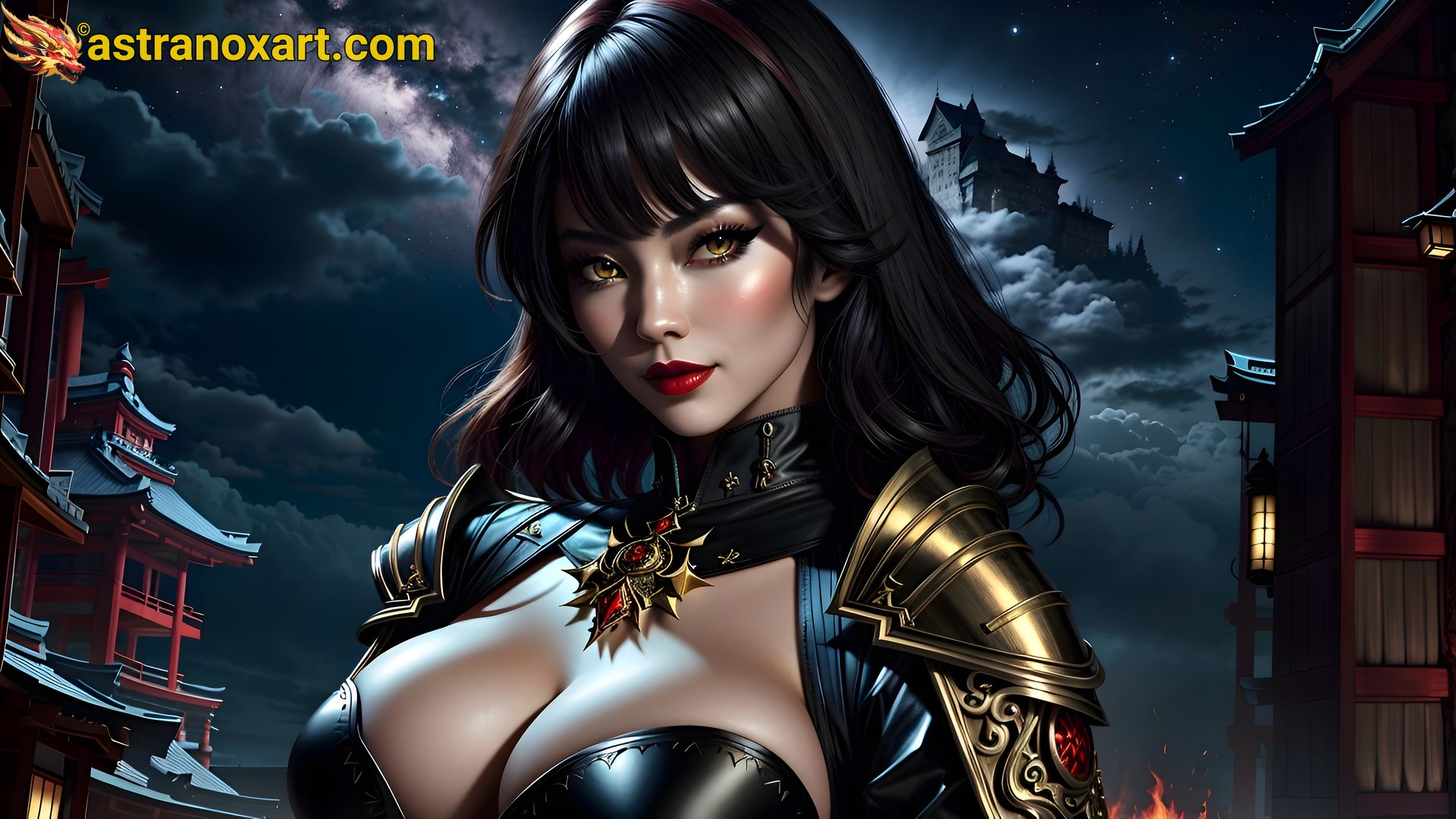The image depicts a striking samurai warlock avatar, an animated young woman with an exotic Asian appearance. She stands in partial profile, gazing seductively at the viewer with golden-colored eyes accentuated by heavy eye makeup and bright red lips. Her straight black hair falls to her shoulders, framing her face elegantly. She is adorned in a tight black leather outfit that barely covers her chest and features a black choker from which a gold and red medallion dangles. Gold or bronze shoulder pads extend into a protective arm guard, enhancing her warrior-like aesthetic. Her large breasts are highlighted by her metal bra, adding to her formidable presence.

The ominous nighttime sky with swirling clouds creates a dramatic backdrop, suggesting a sense of foreboding. Looming behind her is a grand castle in the clouds, emphasizing her mystical surroundings. Flanking her are traditional Asian-style structures, with red, octagon-shaped buildings on either side. In the top left corner, a fantastical red and yellow dragon head along with yellow letters spell out A-S-T-R-A-N-O-X-A-R-T dot com. With its rich detail, this image evokes a scene from an anime fantasy video game, blending elements of ancient tradition and magical realism.